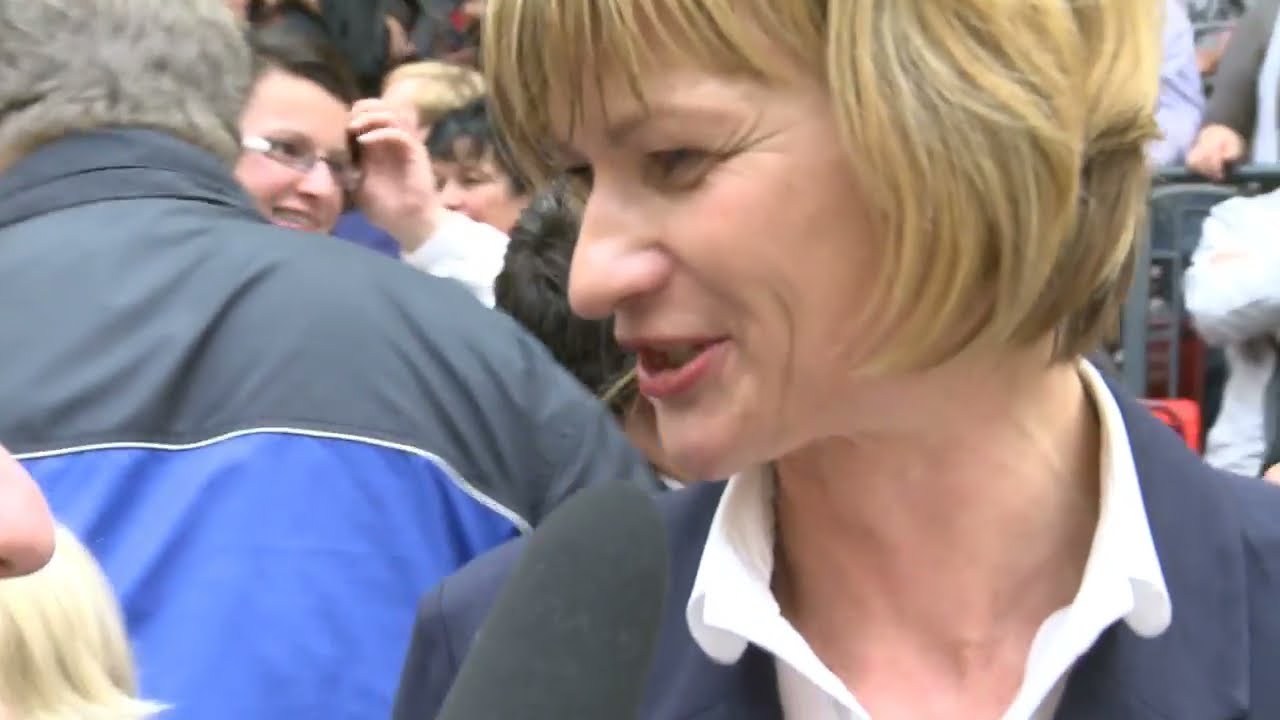This wide rectangular photograph captures a high school basketball game in a bustling gymnasium. The glossy light brown tiles of the court occupy the bottom two-thirds of the image, adorned with white, red, and blue stripes. Both teams are present on the court, with the team in white featuring prominently in the foreground. On the left side of the image, three white-uniformed players are clustered together; two of them have their arms around a third player, supporting him off the court, indicating a likely knee or ankle injury. Two additional players from the white team are positioned on the right side, facing away from the camera. The orange-uniformed team is also visible, with one black player engaging with a white player, while the rest converse among themselves. The upper portion of the image reveals several rows of filled seats, extending from right to left, indicating a sold-out crowd. Various signs are visible at the edge of the seating area, enhancing the impression of a well-attended game.